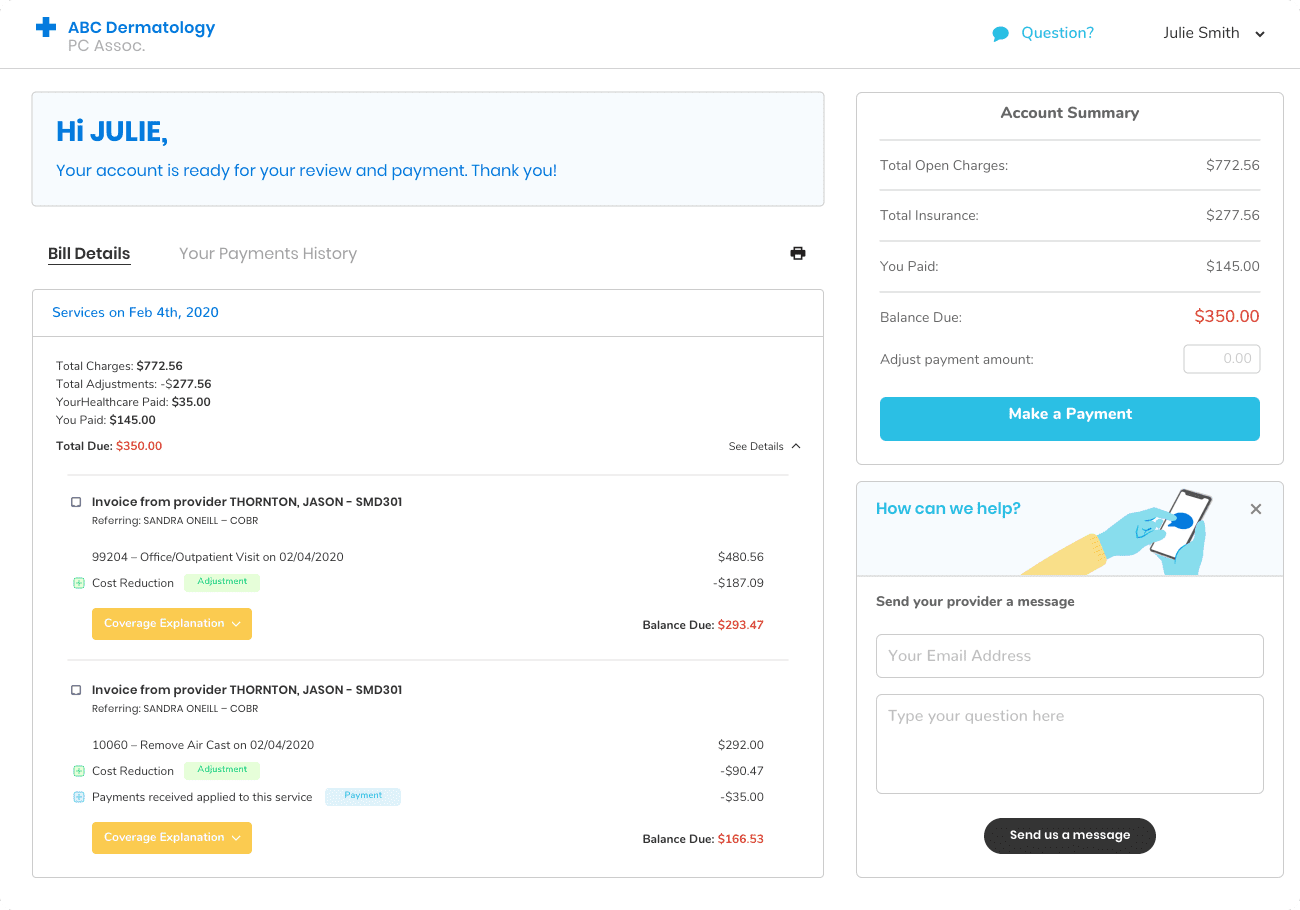### Image Description

The image displays a webpage from a dermatology website viewed on a computer screen, presumably a patient's personal account portal. The entire background is a plain white, employing the default screen color from the user's device.

At the top left corner, there's a blue plus sign followed by the title "ABC Dermatology" in blue font. Beneath that, in gray, it reads "PC ASSOC." Moving horizontally to the right, there is a light blue text of "Question" next to a chat icon. Directly to its right, "Julie Smith" is displayed in black font with an option to click on it.

A thin black line separates the header section from the main content. Below this line, within a light blue box, the text reads, "Hi Julie, your account is ready for you to review and payment. Thank you." 

Following this message, in bold black font, it states "Bill Details." Underneath, in a lighter black or gray font, it reads "Your Payment's History" beside a small print button. The service date included is February 4th, 2020, along with detailed charges and the total amount due. There are clickable options for viewing "Coverage Explanation" and another invoice from "Jason Thornton."

On the right-hand side, the "Account Summary" is summarized in bold black font. Below it, in standard black font, are details such as total open charges, total insurance, payments made, and the remaining balance due. Options are provided to adjust the payment amount and make a payment. There is also a "How can we help?" section for sending messages.